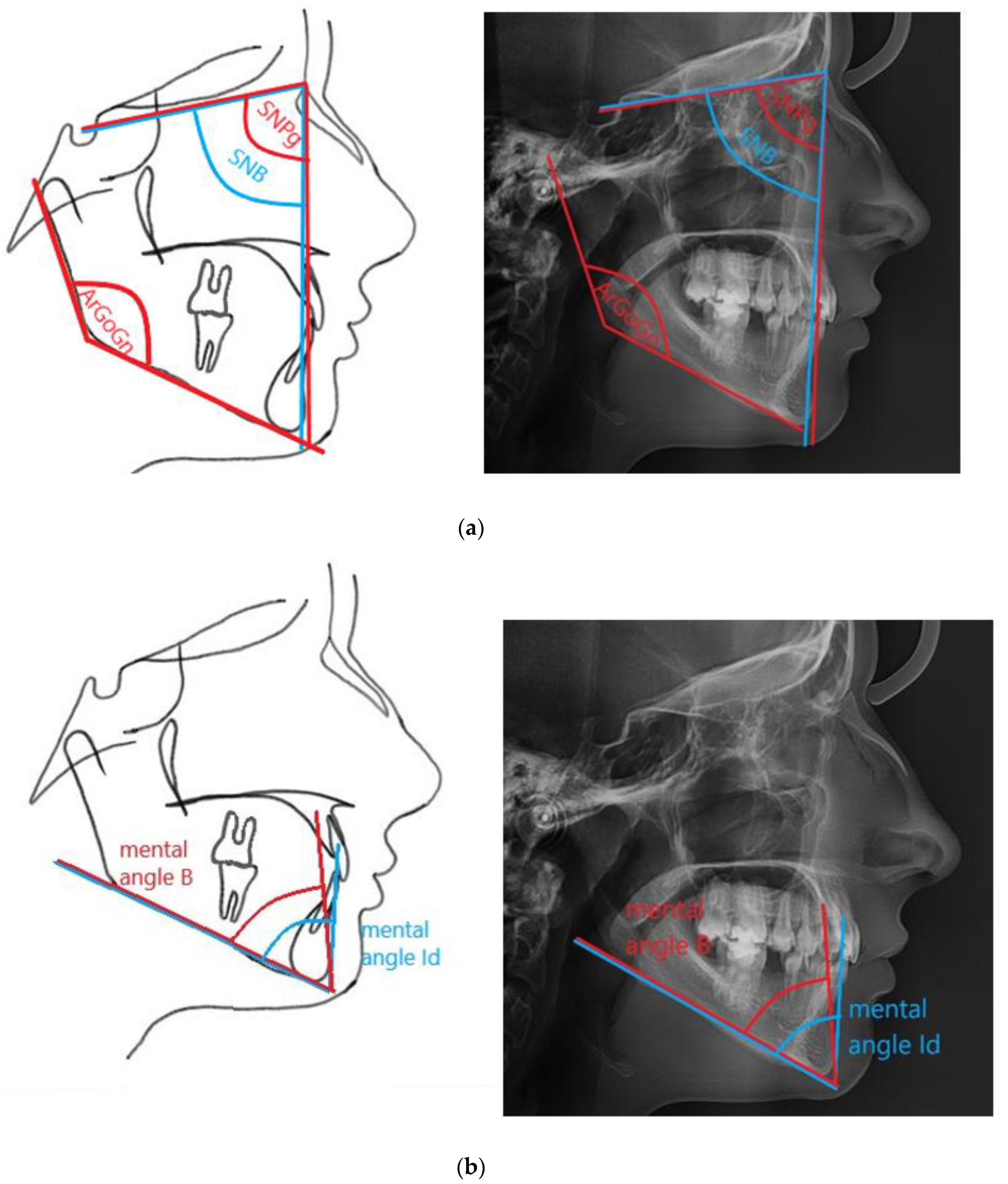The image displays an x-ray of a person's teeth divided into four sections with labels A and B. The left side of each section includes a detailed black-and-white profile illustration of a man's face, highlighting the molar area to the chin with red and blue markings. Annotations include SMPG, SMB, and ARGOGM, alongside text indicating "mental angle B" and "mental angle ID." The right side features corresponding x-ray scans with similar markings, set against a grey image on a black background, characteristic of dental imagery. In section A, red lines trace a trapezoidal path from the ear to the chin and eyes, while section B has a simpler red line pattern extending from the back of the cheek to the chin and nose, with a blue line marking "mental angle ID." This detailed presentation seems to outline potential dental work needed, showcasing both artistic representations and actual x-ray evidence of the individual's dental structure.